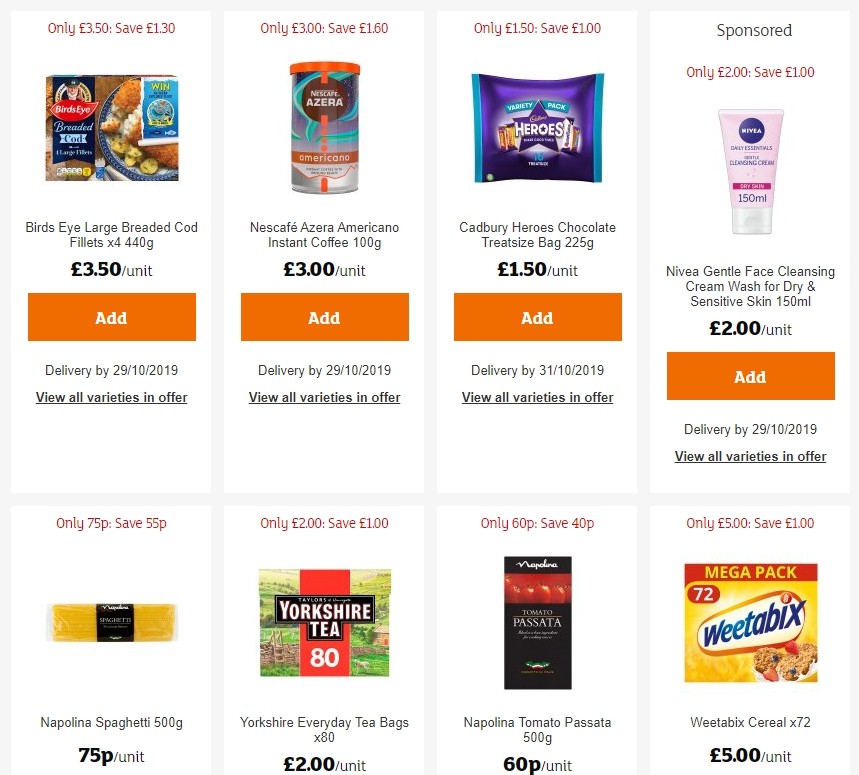This is a detailed screenshot of a grocery shopping app, displayed in English and using British pounds (£) as the currency. The app showcases eight distinct grocery items, each accompanied by its unit price. Below each item, there is an easily identifiable orange "Add" button, which suggests functionality for adding items to an online shopping cart. This feature likely indicates that the app is designed for users to create their grocery orders digitally, possibly for a click-and-collect service where they can later pick up their pre-selected groceries.